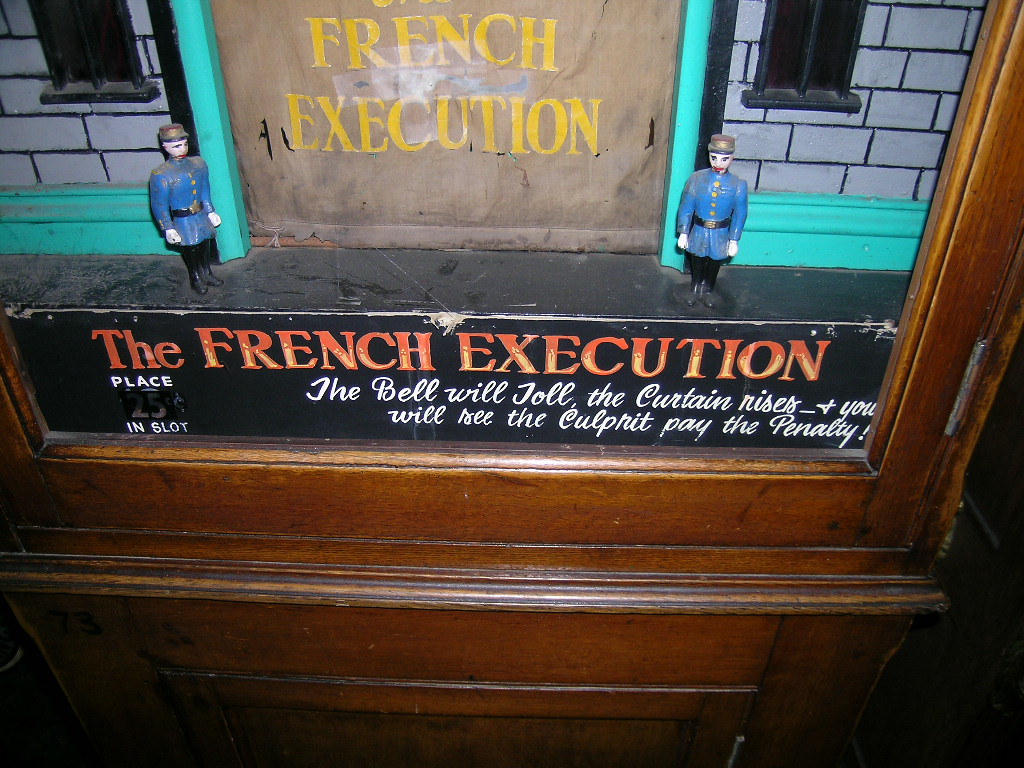This photograph depicts an antique, mechanically-operated slot machine display, housed within a red wooden cupboard, likely found in a museum. The display case features an intricate diorama scene with two miniature French soldiers positioned to the right and left, standing in front of a white brick wall with black jail-like windows. The center of the display showcases a deteriorating brown curtain with yellow lettering that reads "French Execution," framed by a turquoise border. 

In front of the miniatures, a black sign with red text commands attention, reading "The French Execution." Below this, in white cursive lettering, instructions explain, "Place 25 cents in slot. The bell will toll, the curtain rises, and you will see the culprit pay the penalty." This detailed diorama scene, encased behind glass in the wooden cupboard, captures the grim specter of a historical execution, enhancing the viewer's museum experience.